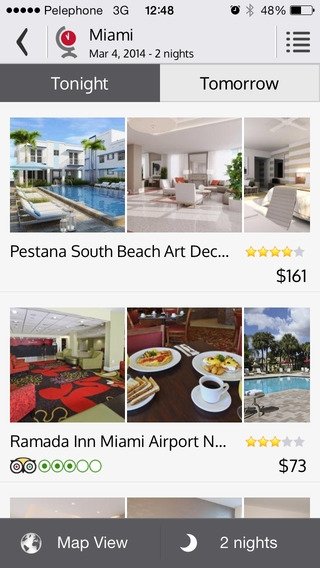A screenshot captures the display of a smartphone, showing someone planning a vacation and evaluating hotel options based on pictures and details. The phone interface displays information at the top indicating a 3G connection, a current time of 12:40 AM, an alarm clock icon, Bluetooth status, and a battery life at 48%. Five vertical bars with dots are also visible on the screen.

The primary content includes details about the trip: "Miami, March 4th, 2014, two nights." The user is comparing hotels, including the "Armada Inn, Miami by the airport." A prominent option featured is the "Masala South Beach Art Deco Hotel," priced at $169 per night, with a second price listed as $161. This hotel boasts a four-star rating.